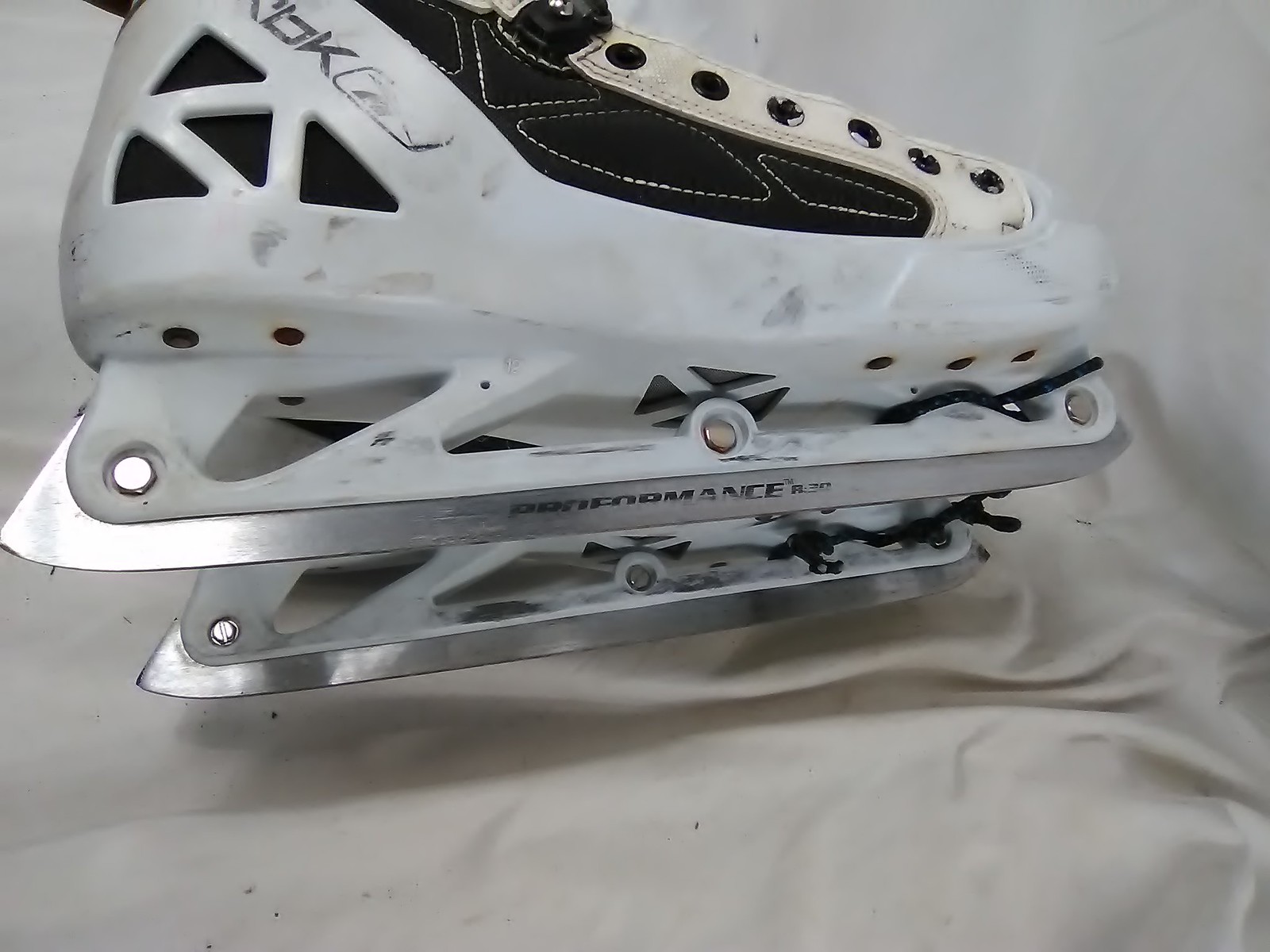This photograph showcases a single ice hockey skate prominently centered on an off-white, crumbled fabric, resembling either a sheet or silk. The skate's boot is primarily white with black accents, featuring notable wear and tear through black smudges and scuffs. Notably, there are four solid black triangular cutouts near the heel. The skate is equipped with two extremely sharp blades, visibly secured by three silver bolts on the right side, and bears the text 'Proformance R30' in black letters on the blade. The lace holes are conspicuously empty, and above them, there is a black Velcro strap. Only one skate is fully visible, with the other partially obscured behind it.